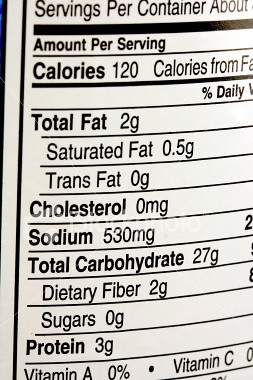A close-up image displays the back label of a food product, showcasing detailed nutritional information. The white label features black printed text that begins with "servings per container about" (the exact number is not visible). The nutritional facts per serving are listed as follows: 120 calories, 2 grams of total fat, 0.5 grams of saturated fat, 0 grams of trans fat, 0 grams of cholesterol, 530 milligrams of sodium, 27 grams of total carbohydrates, 2 grams of dietary fiber, 0 grams of sugars, and 3 grams of protein. At the bottom, there is a breakdown of percentage daily values for certain vitamins, although the specific vitamins and corresponding percentages are not clearly visible. The product identity remains unknown based solely on this label information.